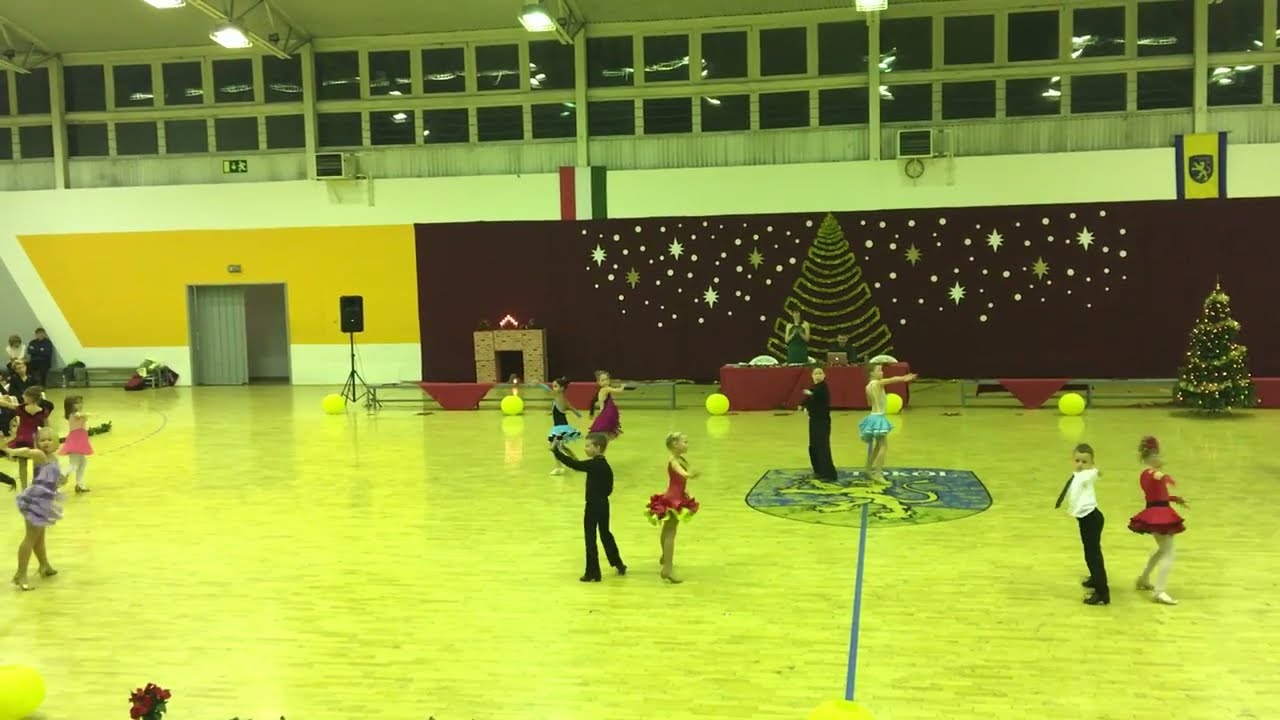In the image, we see an indoor scene set in a large gymnasium with a hardwood floor that features a prominent logo, resembling a crest or a lion banner, at its center. The central focus of the image is on several pairs of children, boys and girls, dancing in what appears to be an old-style dance, possibly the cha-cha. The boys are dressed in button-up shirts, some with ties, while the girls wear dresses. 

The backdrop of this festive scene is adorned with Christmas decorations, including gold trees, stars, and what looks like a fake fireplace. Red tables are set up in the background, near which a woman in a green dress stands. Additionally, there is a man at a laptop, likely controlling the music, with speaker stands positioned nearby. 

The gymnasium walls are painted yellow and purple, and display two national flags. High up on the walls near the ceiling, there are large glass windows. This indoor event, likely taking place in the evening, appears to be a formal dance or perhaps a lesson in ballroom dancing.